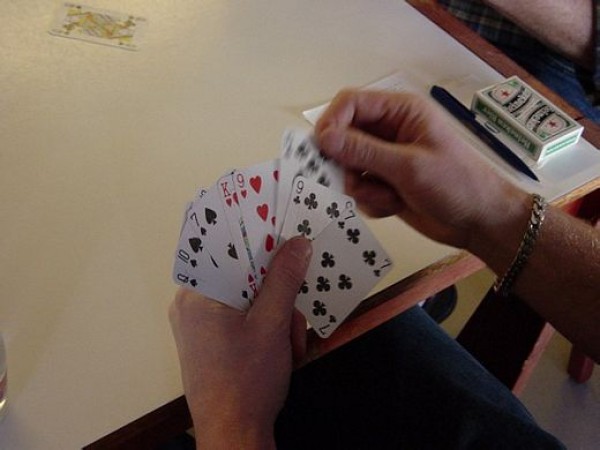This is a vivid color photograph capturing a moment where a man is engaged with a deck of playing cards. Only his hands and a part of his legs are visible. His left hand holds the cards fanned out, while his right hand hovers as if about to select one. He wears a gold chain bracelet on his wrist, which adds a touch of elegance to the casual scene. His knee, clad in what appear to be blue jeans, protrudes slightly from the bottom left of the frame. The setting includes a brown wooden table covered with a white tablecloth. In the upper right corner of the image, the box that originally housed the cards is visible, along with a slender black marker or felt-tip pen. The upper left corner shows a slightly out-of-focus face card, though its rank and suit are indeterminate. The lower right corner reveals a small section of the floor, which is a subtle slate blue color.